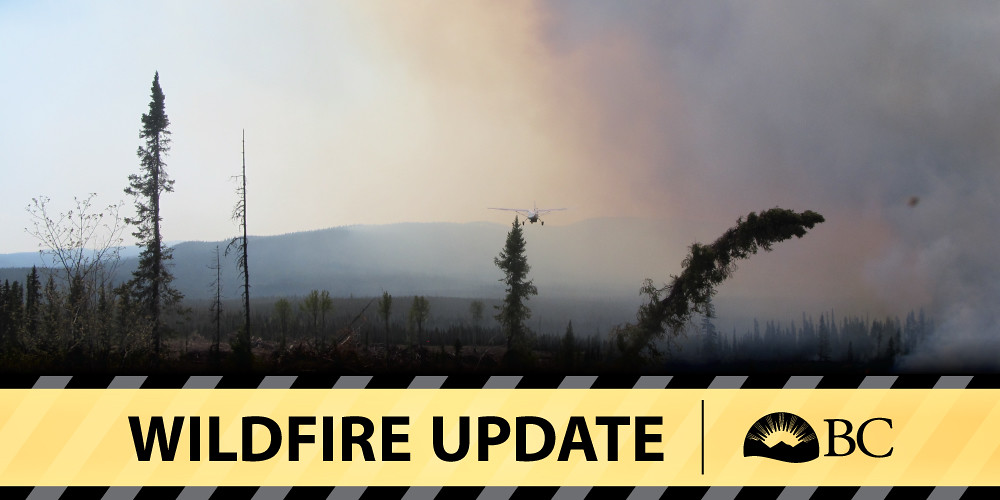The image portrays a wildfire raging in a valley nestled between two hill ranges. The foreground features a few spindly trees standing amidst sparse grass. The left-hand side of the photograph shows more trees, while the right-hand side is dominated by thick smoke, tinged with an orange hue at the bottom, indicating the fire’s location. In the center of the image, a small white propeller plane is visible, flying just outside the dense smoke. The scene is overlaid with a yellow bar containing a “wildfire update” notification in black text, accompanied by a rising sun and mountain logo with the letters "BC." Diagonal white bars decorate the notice, enhancing its visual appeal.